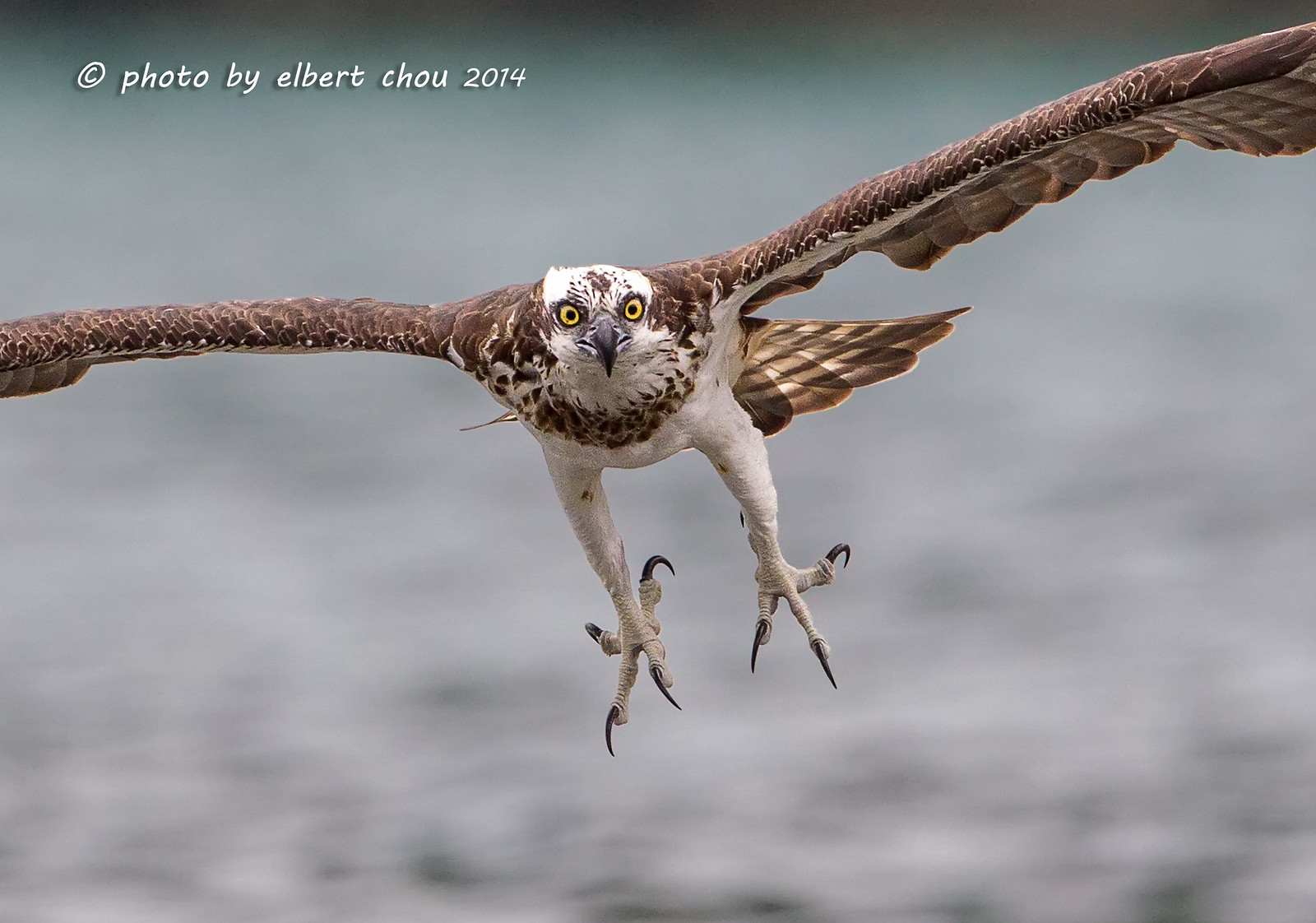This full-color photograph, taken during the daytime in 2014 by Albert Cho, captures a majestic bird of prey, likely a hawk, soaring over a body of water with a blurry blue backdrop. The hawk, with its large wings fully extended, is in mid-flight, looking directly into the camera with striking yellow eyes that have dark centers. The bird’s plumage features a distinctive combination of brown wings and tail, a white head, chest, and legs. Its sharp talons are extended and ready to grasp its next target, indicating a predatorial stance. The image, marked with a note at the top left corner attributing it to Albert Cho, encapsulates the powerful and dynamic essence of the hawk in motion.